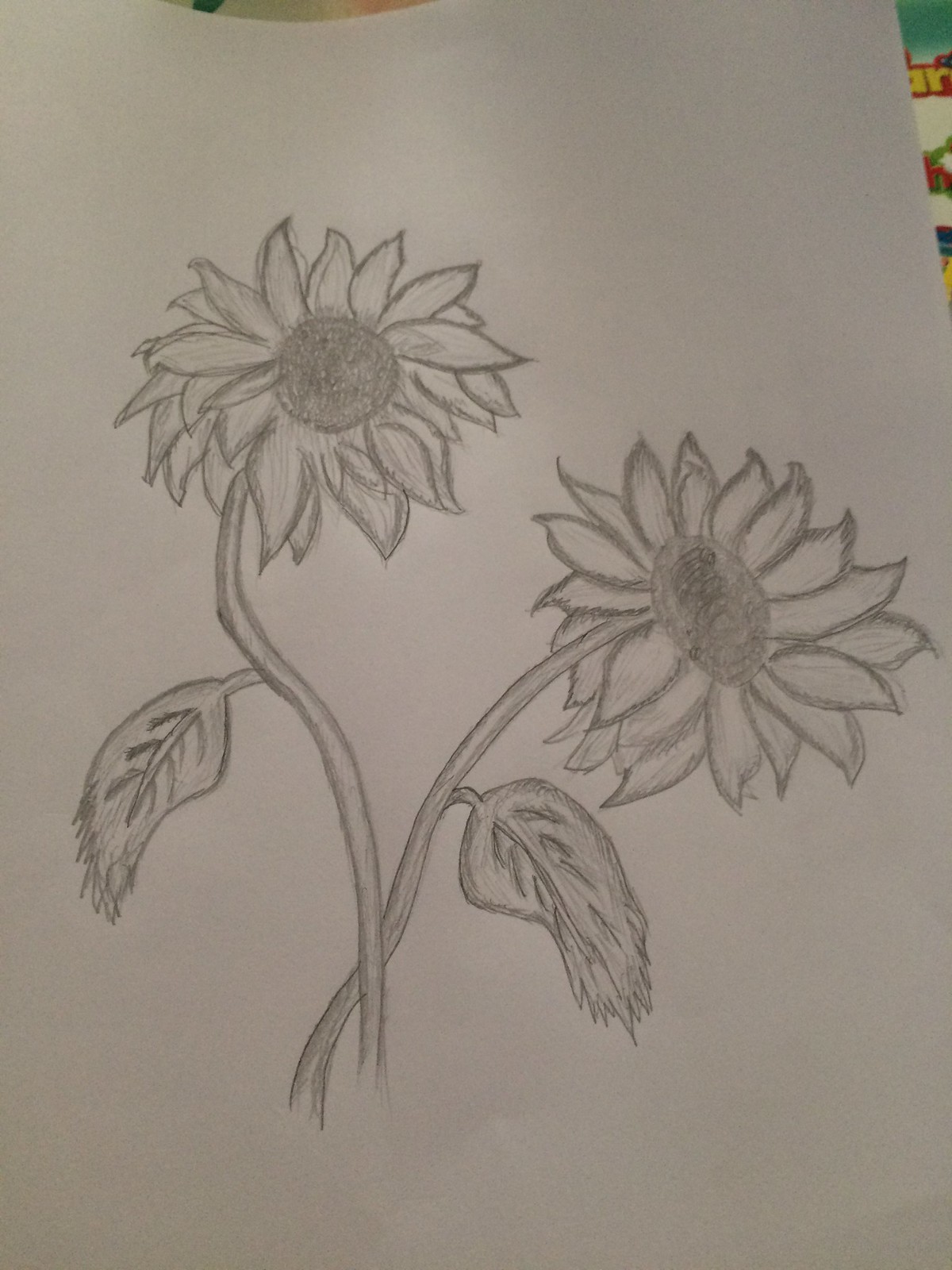A meticulously detailed pencil illustration on white paper showcases the stems and flowers of red sunflower-like blooms. The left stem supports a flower with numerous petals, 20 or more, each intricately shaded with dark pencil edges. A solitary leaf protrudes from the left side, characterized by frayed edges and a pronounced veiny structure. The right side of the drawing features another flower and similarly detailed leaf structure. Both flowers exhibit densely packed petals surrounding a dark, textured center. The entire piece is shaded with a careful hand, emphasizing the natural beauty and complexity of these floral elements.